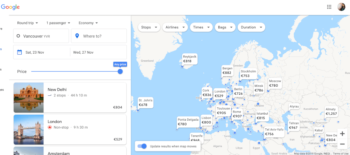This image appears to be a small, pixelated screenshot from the Google website, featuring a travel planning interface. In the top left corner, the recognizable Google logo is visible. Dominating the right side of the image is a large map displaying Europe and various regions of the Middle East. The map showcases distinct sections and labels, likely including names and prices, indicative of travel destinations. The map itself uses a blue color to denote oceans and white for the landmasses, creating a clear contrast.

On the left side of the image, there are options that allow users to select travel dates, including start and return dates. Additionally, photos of various destinations are present in the bottom left corner, though they are quite small and blurry. One of the destinations is mentioned to be London, but the text is not clearly readable due to the low resolution.

The entire website is displayed in a white mode, giving the background a clean, white appearance. In the top right corner of the image, there seems to be a dark-colored circle or sphere, although its purpose is unclear from the context provided in the screenshot.